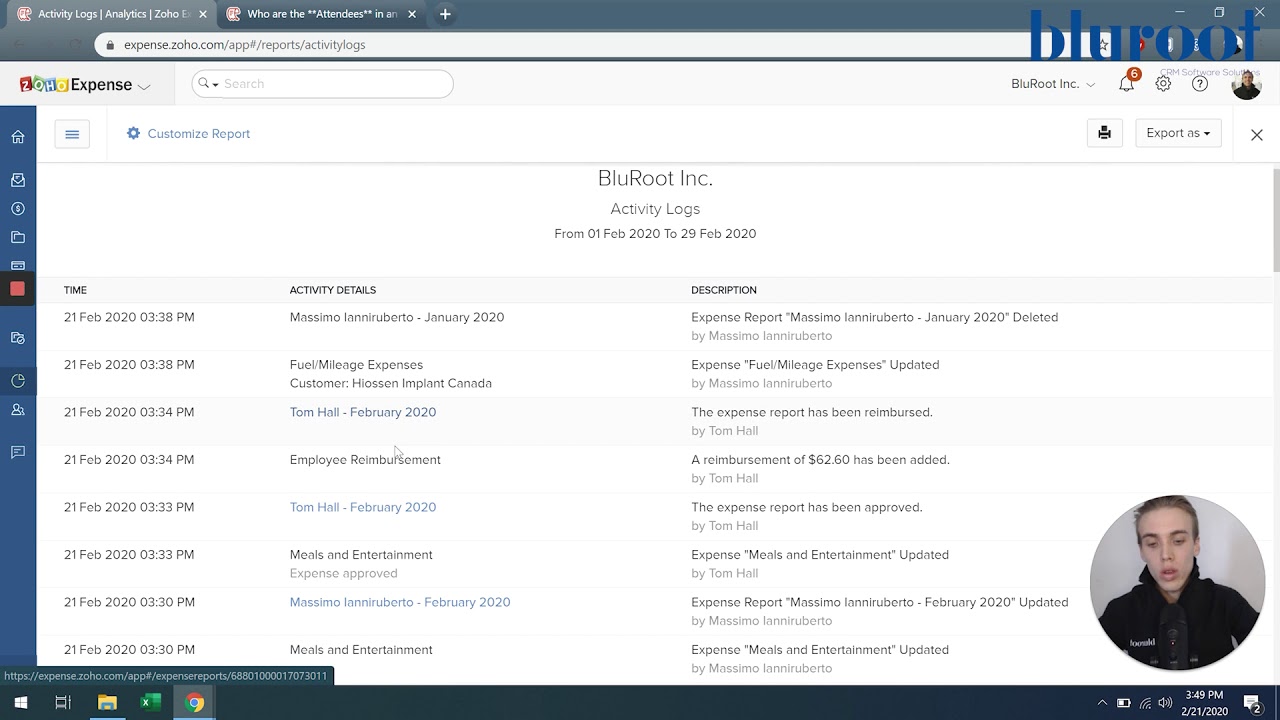The image depicts a screenshot of a website interface. At the top right corner, the text reads "Blue Root," followed by a colorful block that says "ZOHO" on the left and "Expense" inscribed in black lettering. Below, several columns are visible with a title "Custom Report." The central part of the screen displays the heading "Blue Root, Inc. Activity Logs from 01-Feb-2020 to 29-Feb-2020," arranged in three columns: Time, Activity Details, and Description, all labeled in black. The time column lists dates and times, starting with an entry on 21-Feb-2020 at 03:38 pm. Underneath, one can see the activity details and corresponding descriptions for eight expense reports.

In the lower right-hand corner, there is a circular icon with a gray background featuring an image of a young man. He wears a black jacket, looks downward while facing forward, and has slicked-back hair of medium color. The bottom of the screen is bordered by a black strip showcasing some computer buttons. On the left side of this black border, the current time and date are displayed.